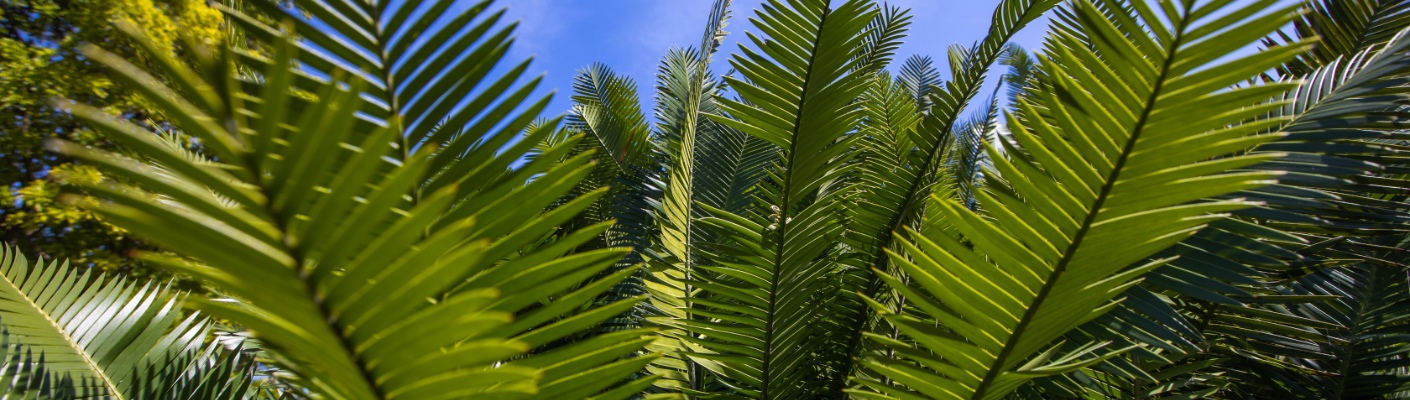A panoramic shot captures a dense field of lush, fan-shaped foliage stretching across the image like a verdant banner. Dominating the foreground are numerous clusters of long, slender leaves, each with brown stems and myriad smaller fronds radiating outward like miniature palms. These plants, numbering over twenty, form a verdant canopy, obscuring the view of their bases and creating a sea of green fans that seem to be floating in mid-air. On the left, partially hidden by the predominant foliage, is a distinct, bushier plant, its verdant presence just peeking through the dense leaf cover. Above, the sky peeks through this leafy expanse, a brilliant blue canvas adorned with delicate, wispy clouds, adding a serene backdrop to the botanical display.